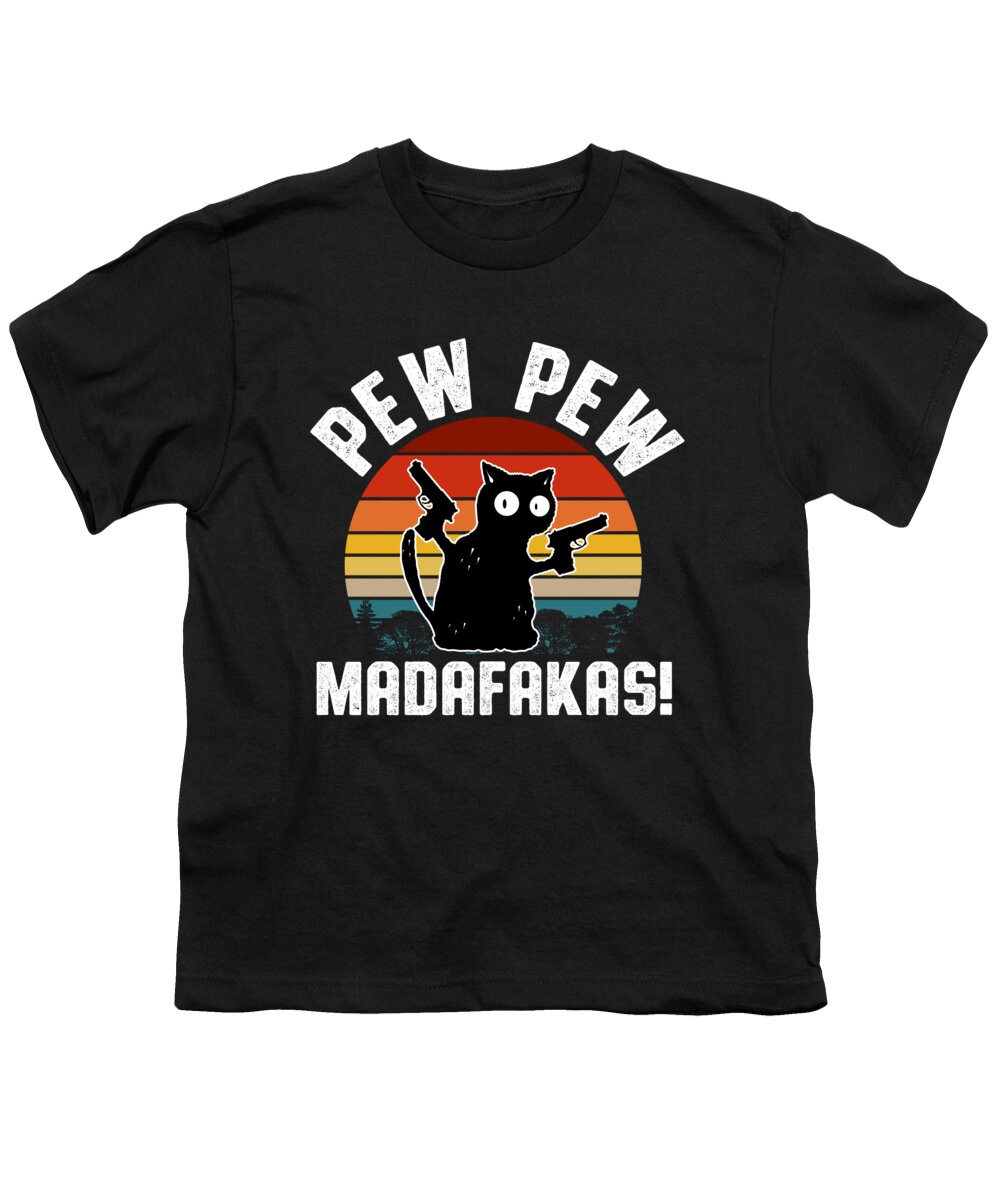This detailed product image is a color photograph of a black short-sleeved t-shirt with a round crew neck, likely suitable for e-commerce platforms like Teespring or Redbubble. The t-shirt features a humorous and eye-catching graphic on the front at the chest area. The main element of the design is a stylized sunset, represented by a circular motif with horizontal stripes that transition through various shades of red, orange, yellow, beige, and blue, culminating in a green stripe at the bottom that suggests a landscape with trees.

Overlaying this vibrant backdrop is a cartoonish black cat with wide white eyes, humorously clutching a pistol in each paw. The feline appears to be sitting up, looking back over its right shoulder. Above the cat, bold white text exclaims "PEW PEW," while below the circle, the phrase "Madafakas!" is written in a similarly bold style, stylized as "MADAFAKAS!" with an exclamation point, adding a cheeky and irreverent twist to the design. The overall style of the graphic blends elements of photographic realism and representational art, making for a unique and amusing t-shirt design.